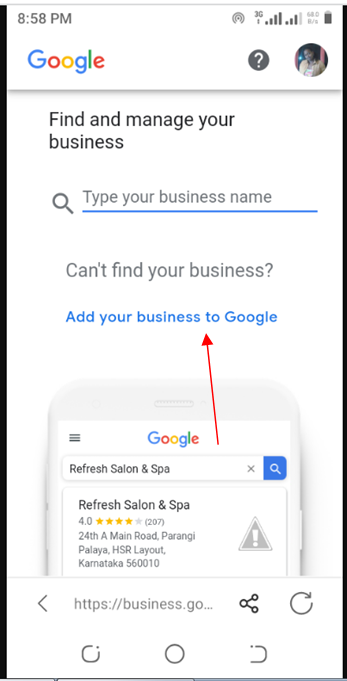A detailed screenshot description of a user's phone:

In this screenshot, the user is on a Google search interface displayed in a light theme. The "Google" logo is prominently positioned on the top left corner. On the top right corner, there is the user’s profile picture. Between the Google logo and the profile picture, there is an interactive help icon marked with a question mark.

Below the header, the text "Find and manage your business" is repeated twice. The search bar is displayed with a magnifying glass icon on the left, next to a vertical blue line where users can input their search terms. Currently, the search bar is empty, and no business name has been entered.

Below the search bar, there's a prompt that reads "Can't find your business?" followed by a call-to-action link, "Add your business to Google". Alongside this text, there is an illustration of a smartphone displaying a guide on how to add a business to Google. The example business shown in the phone illustration is "Refresh Salon and Spa", complete with search entry and associated details like the address.

Immediately below the illustration, search results for "Refresh Salon and Spa" are displayed, including the business details and a link to its webpage. To the right of the business information, there is a share icon depicted by three connected circles forming a triangle. Beside the share icon is a refresh icon.

At the bottom of the screenshot, the typical phone navigation menu is visible, featuring the back, home, and recent apps buttons commonly found on most smartphones.